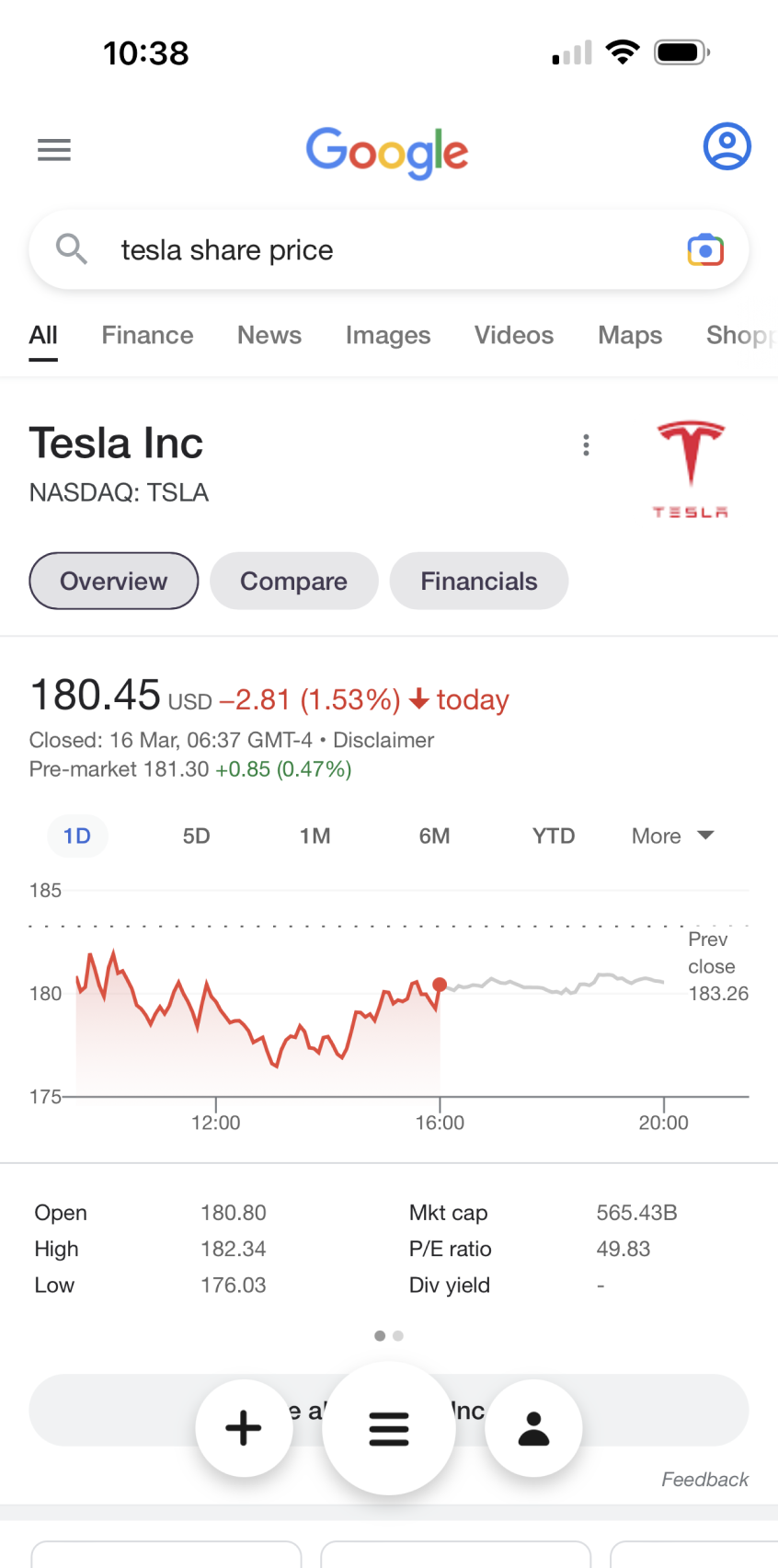**Detailed Caption:**

This mobile screenshot showcases a Google search result for Tesla's share price. The background is predominantly white, with the distinctive Google logo prominently positioned at the top center. Adjacent to the Google logo on the right is a blue user profile icon, while a black menu icon is located at the far left.

A long search bar stretches almost entirely across the top, containing the query "Tesla share price" in small black lettering. Directly beneath the search bar is a horizontal navigation row with various categories like All, Finance, News, Images, Videos, Maps, and Shopping, with "All" being the selected option.

The main search results begin just below this row. "Tesla Inc" is displayed in large black font, followed by "NASDAQ: TSLA" in bold grey text. On the right side of the page near the top, the Tesla logo is visible. Below the logo, there are options labeled "overview," "compare," and "financials," with "overview" currently selected.

In the center of the screenshot, prominently displayed, is the share price "$180.45 USD". To the right of this price, in red font, is the percentage change "-2.81%," with an additional note in parentheses stating "1.53% down today." Further below, it indicates "Closed 18 March 6:37," accompanied by the word "disclaimer" in small grey letters. Below this, it mentions "pre-market price."

At the bottom of the screenshot, a line graph is displayed, providing a visual representation of the stock's performance. A row of dates is situated at the top of the graph, with "One Day" selected. At the bottom of the graph, detailed metrics such as the opening price, high, low, mid cap, and PE ratio are shown.

Finally, at the very base of the screen, there is a row of navigation icons consisting of a small white circle with a plus sign, a larger central white circle with a menu icon, and a white circle with an account sign on the right.